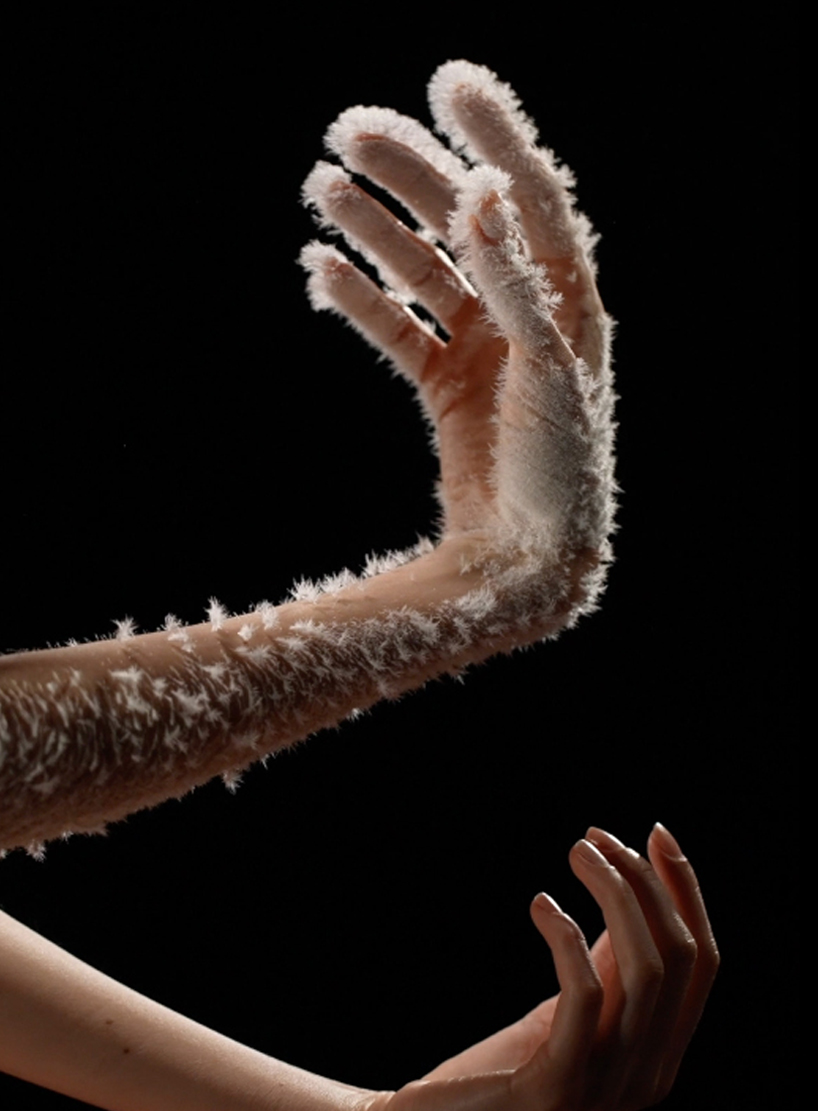In this image set against a stark black background, two hands extend from the left side of the scene. The lower hand, emerging from the bottom left corner, is tan in color and positioned palm-up with fingers loosely curled, as if ready to hold something. Above it, another arm arches in an L shape. This upper hand is notably covered in a dramatic, surreal layer of what appears to be frost or snowflakes, creating an impression of icy feathers clinging primarily to the fingers and less so to the palm and arm. The stark contrast between the normal, light-skinned lower hand and the frosted upper hand, both seemingly belonging to a white woman, adds an element of visual intrigue, heightened by the mysterious, possibly computer-generated nature of the frost-like texture.